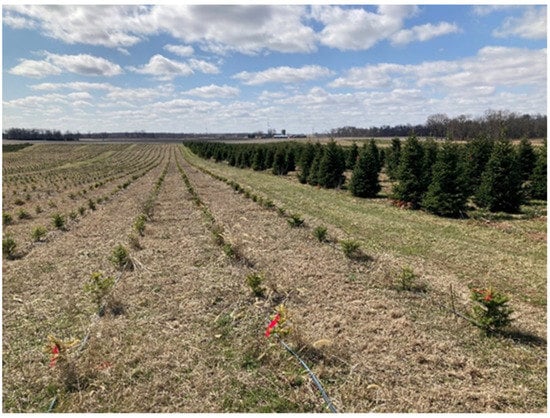This photograph captures an expansive Christmas tree farm stretching toward the horizon under a light blue sky dotted with scattered white clouds. From a central vantage point within one of the many organized rows, the perspective leads the eye down the uniform gaps where young pine trees are neatly planted several feet apart. The trees align meticulously in rows that extend endlessly, seemingly merging at the distant horizon. In the immediate foreground, the earth appears slightly barren, with tufts of dried grass interspersed. Red ribbons mark some of the closest trees, hinting at their readiness for harvest, and delicate wires possibly part of an irrigation or stabilization system crisscross the ground. On the right side of the field, a denser cluster of fully grown, richly green pine trees stands, adding contrast and depth to the scene. In the far distance, a faint outline of a building and a larger forest subtly breaks the horizon, adding further context to this vast and methodically cultivated landscape.